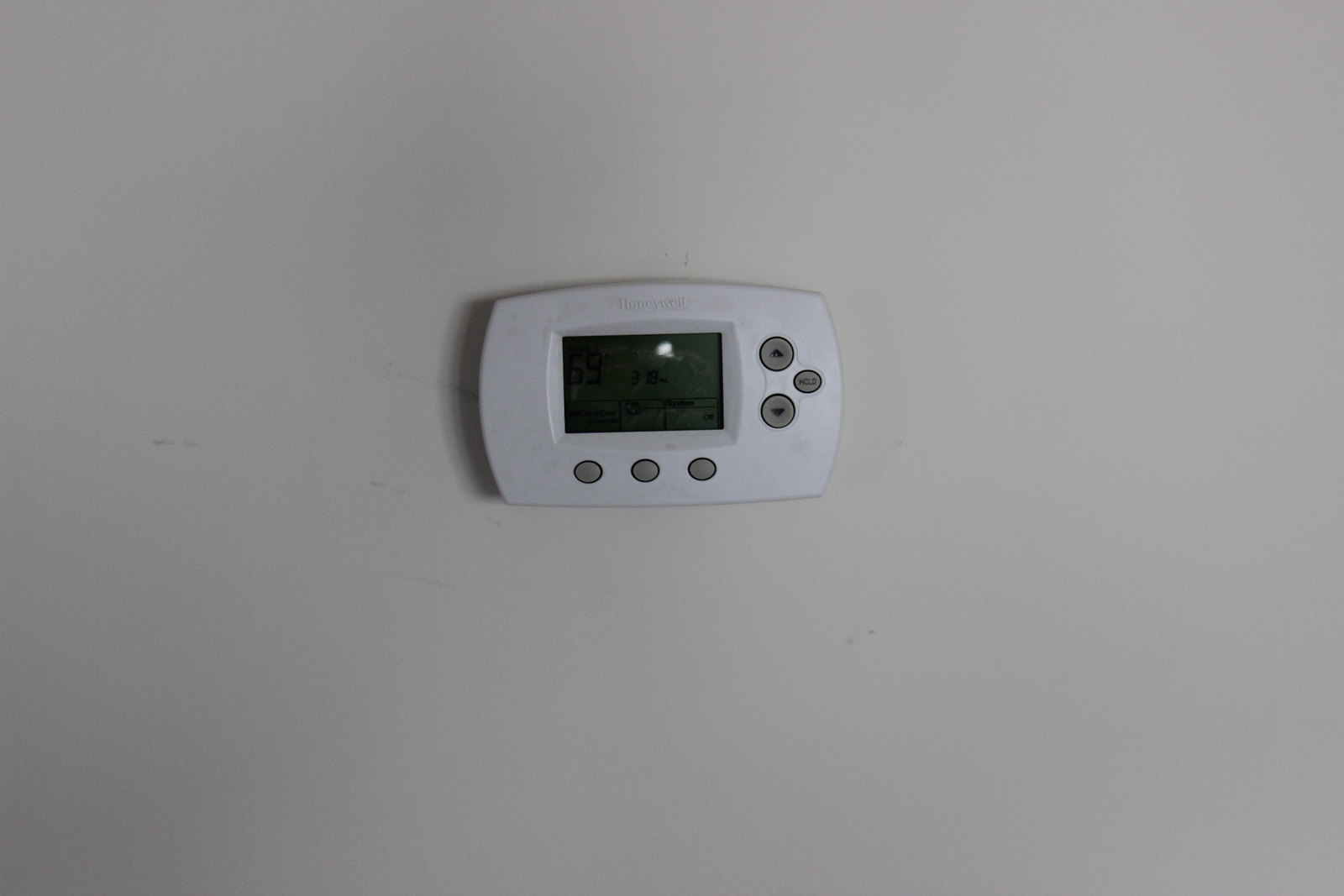A modern, rectangular thermostat with curved edges is securely mounted on a pristine white wall. This sleek, white device features a substantial, slightly recessed LCD display at its center, occupying approximately two-thirds of the thermostat's surface area. Although the brand name, positioned at the top of the unit, is not visible, the functional elements are clearly distinguishable. To the right of the display are two arrow buttons—one for increasing and one for decreasing the temperature—alongside a single "hold" button. Below the screen, three evenly spaced buttons provide additional control options. The overall design, marked by its clean lines and subtly contoured corners, reflects a standard yet contemporary aesthetic.